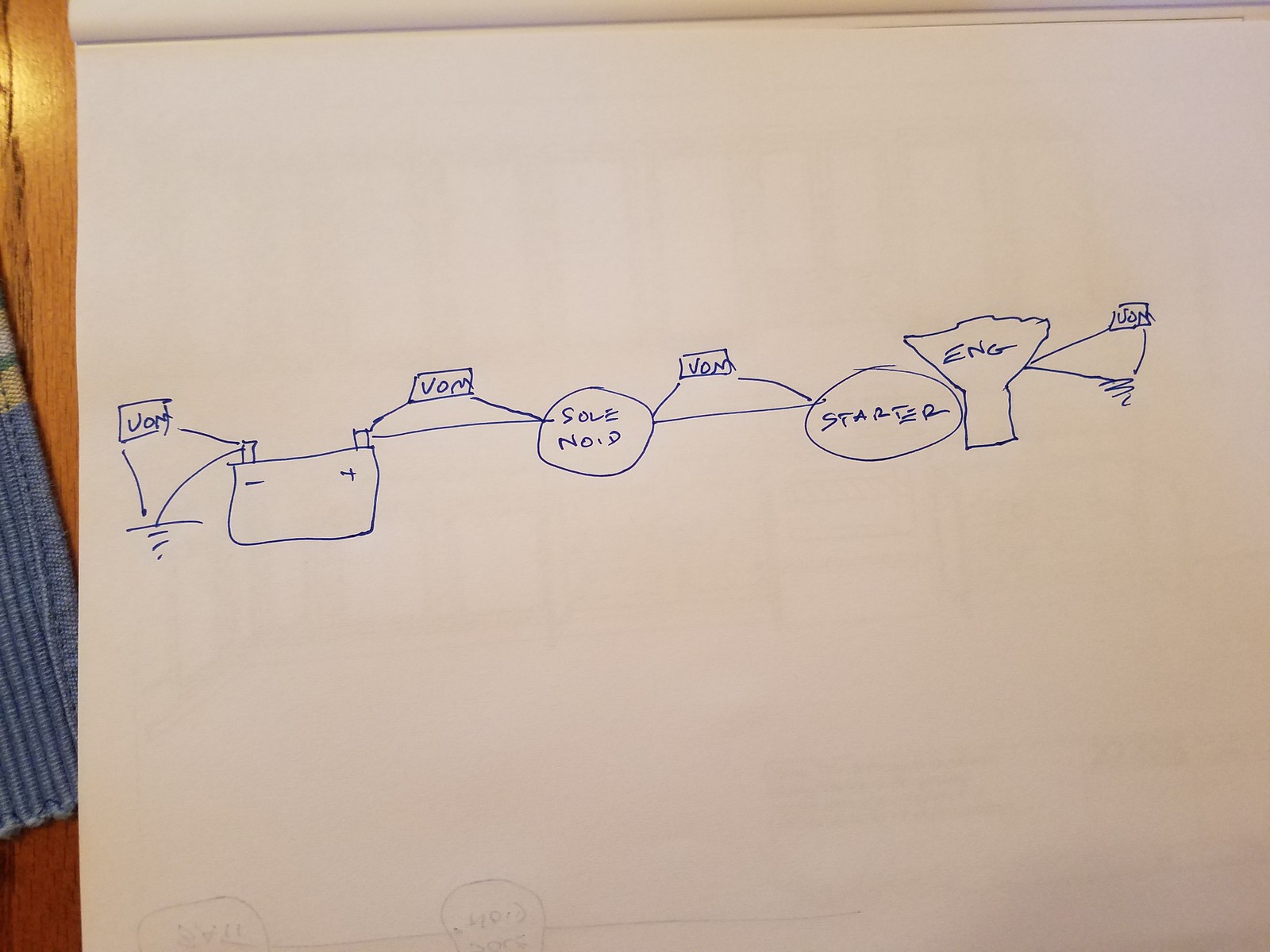This photograph captures a detailed sketch, reminiscent of a schematic diagram, likely outlining an electrical system. The drawing appears to be part of a sketchbook or notepad, as pages are top-bound. The background consists of a wooden surface, possibly a table or wall, accompanied by a blue dish towel adorned with yellow, green, and off-white stripes.

The sketch is rendered in pen and includes multiple labeled components. Several rectangles, each inscribed with "VOM" (possibly referencing a Volt-Ohm Meter), are interconnected by lines to various parts of the system. One "VOM" is linked to the negative terminal of a battery, while another connects to both the positive terminal and a labeled circle denoted as "solenoid." Additional "VOM" rectangles are connected to a "starter" circle and a funnel-shaped symbol labeled "ENG," likely standing for "engine."

The intricate web of connections suggests an attempt to illustrate the flow of electricity or the operation of an electrical circuit, offering an insightful glimpse into the mechanics of the system.